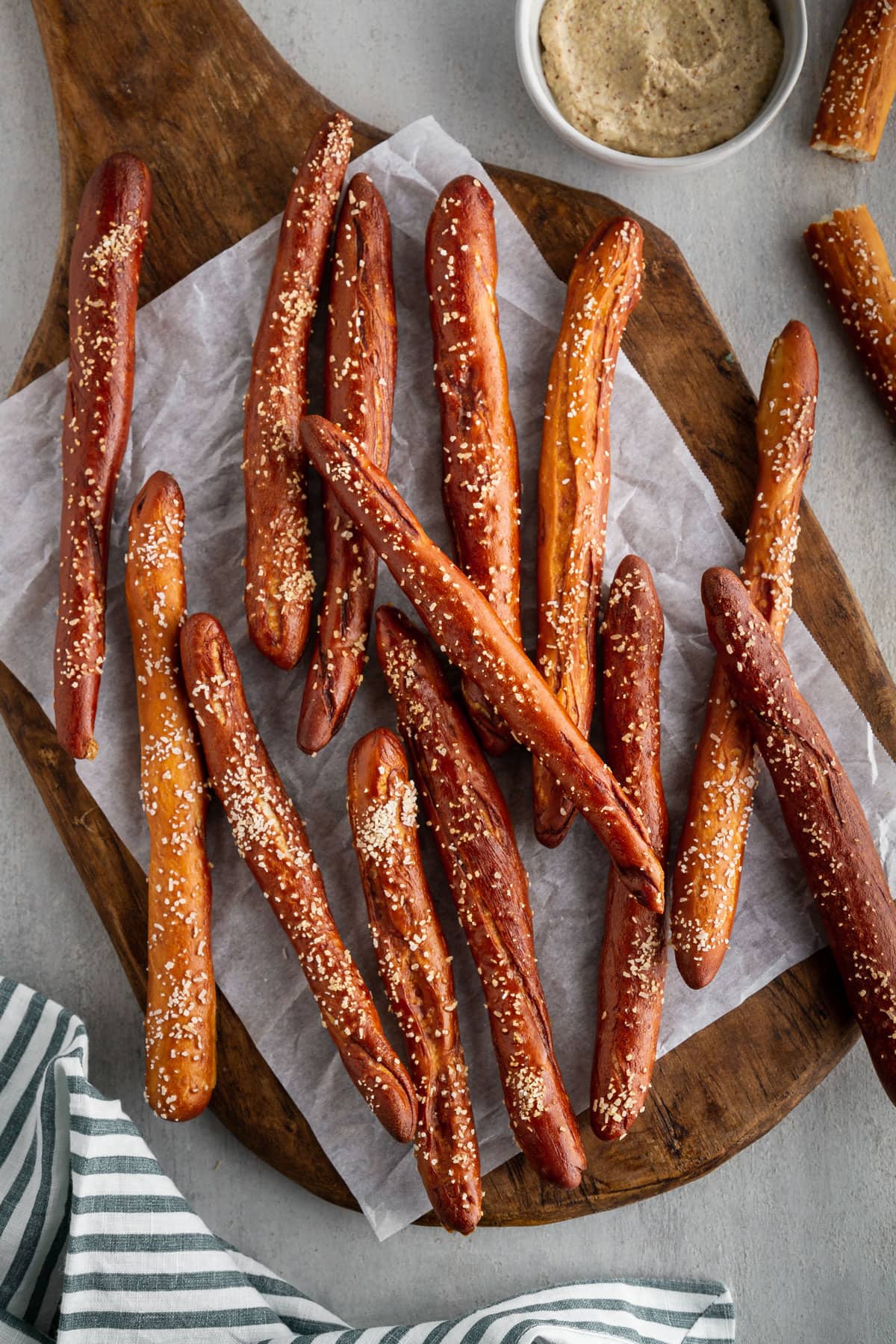The image features a carefully arranged serving of thick, handcrafted pretzel sticks on a wooden cutting board. These pretzel sticks, resembling the size and width of cigars, display a rich pretzel brown hue, indicating they have been well-baked. Each stick is generously sprinkled with coarse salt, noticeable through the numerous white specks on their surface. The pretzels rest on a piece of translucent wax paper, adding a rustic touch to the presentation. Positioned at the top right corner of the board is a small white bowl filled with grainy, handcrafted mustard, serving as a dipping sauce. The setting, likely a restaurant, includes a blue and white striped towel positioned at the bottom left, suggesting a place for diners to wipe their hands. The various colors in the image—pretzel brown, darker browns, gray-green, yellowish-white, and gray—enhance the appetizing and authentic feel of this culinary display.